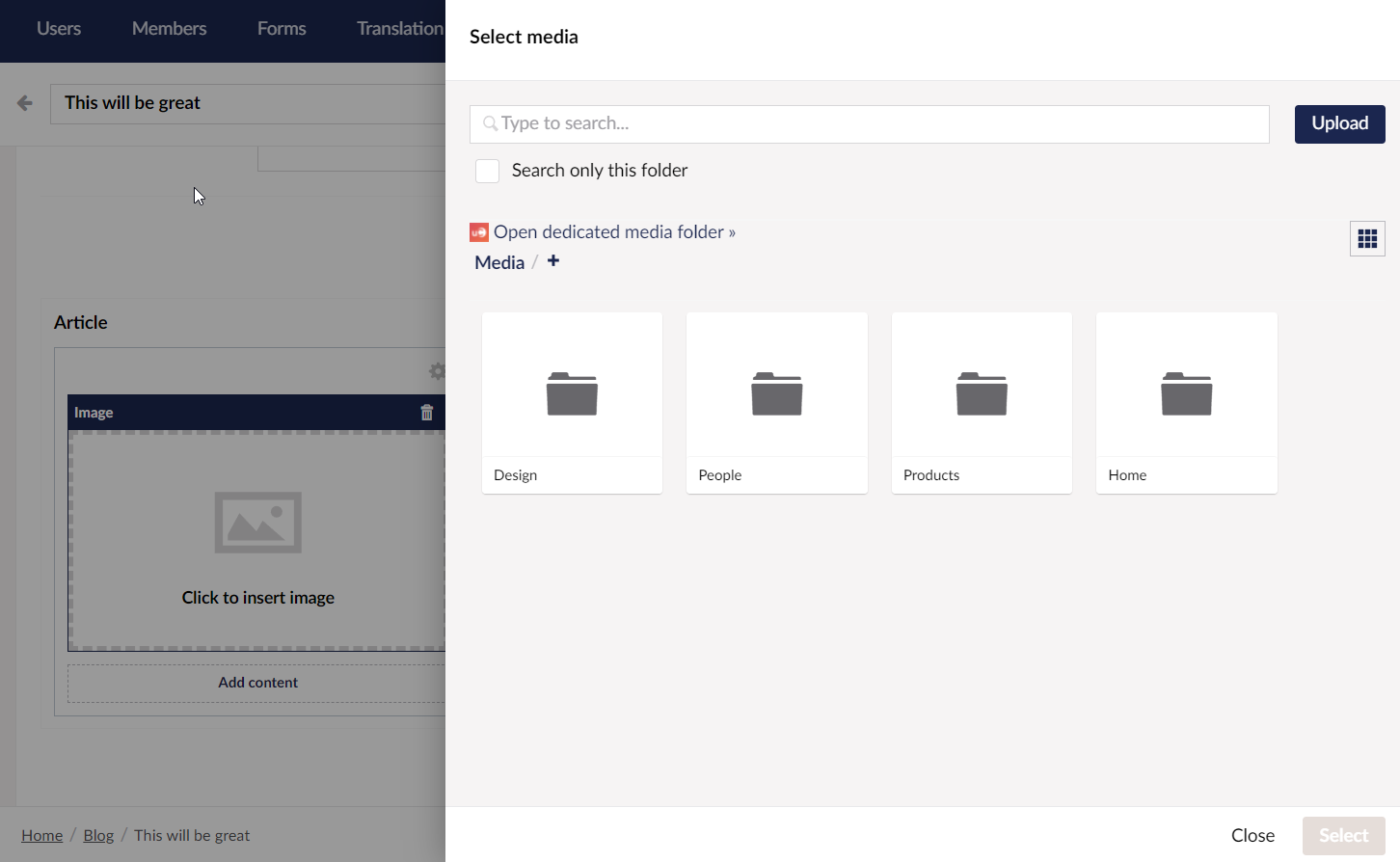**Detailed Caption for Image:**

This image displays a split-screen view of a digital interface, merging elements from both a smartphone and a computer screen. On the left side, the display is predominantly grayed out, with a stark black banner at the top containing navigation options: "Users," "Members," "Forms," and "Translation." Immediately below this banner is a search bar with the placeholder text "This will be great."

Further down the grayed-out left section, a black banner labeled "Image" appears within a square, indicating a placeholder for an image, under a smaller heading that reads "Article." Beneath this, the interface includes an option labeled "Add Contact." In the bottom-left corner of this segment, a breadcrumb trail displays "Home / Blog / This will be great."

Shifting focus to the right side of the screen, a light gray section features the heading "Select Media" at its top. Directly under this, there is a search bar and an upload button. Below this are four white squares, each representing a different media category with a file icon: "Design," "People," "Products," and "Home." At the bottom right corner of this area, there are a close button and a tan button labeled "Select."

An additional red button labeled "Open Dedicated Media Folder" with the path "media \ plus" provides further navigation and organization options for media files.